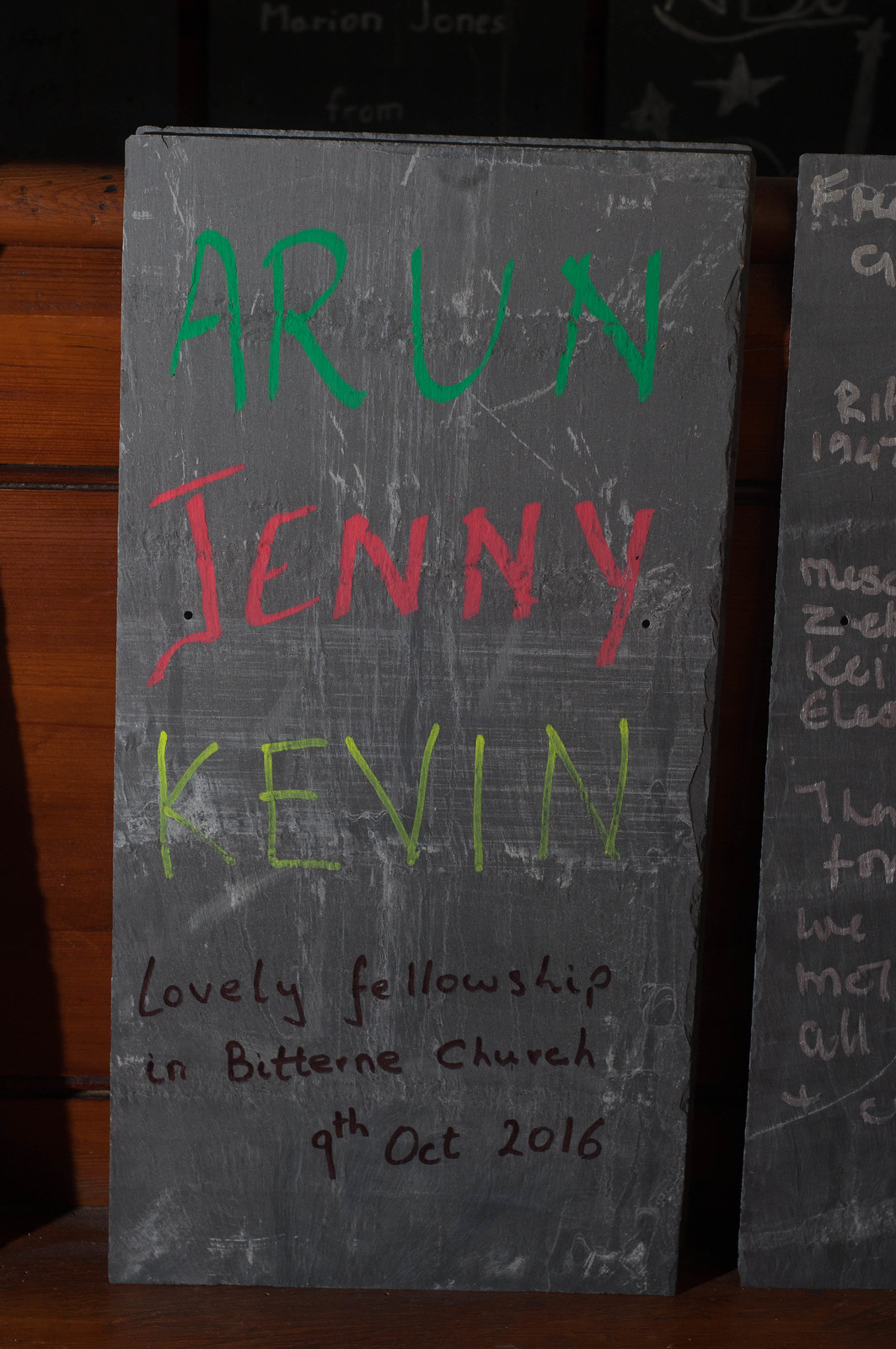The image depicts a dark black sandwich board, possibly coated with chalk paint, positioned on the seat of a wooden bench and leaning against the backrest. The board is scratched and marked, suggesting frequent use. Written on it in various colors of chalk are the names and details: "A. Run" in green, "Jenny" in red, "Kevin" in yellow, and below these, in black lettering, reads "Lovely Fellowship in Bittern Church, 9th of October 2016." Adjacent to this board, there is a similarly colored and sized board with white chalk writing, but only about four inches of this second board is visible due to the image's framing. The scene is well-lit with natural light, revealing a wooden structure in the background, possibly the bench or a wall.